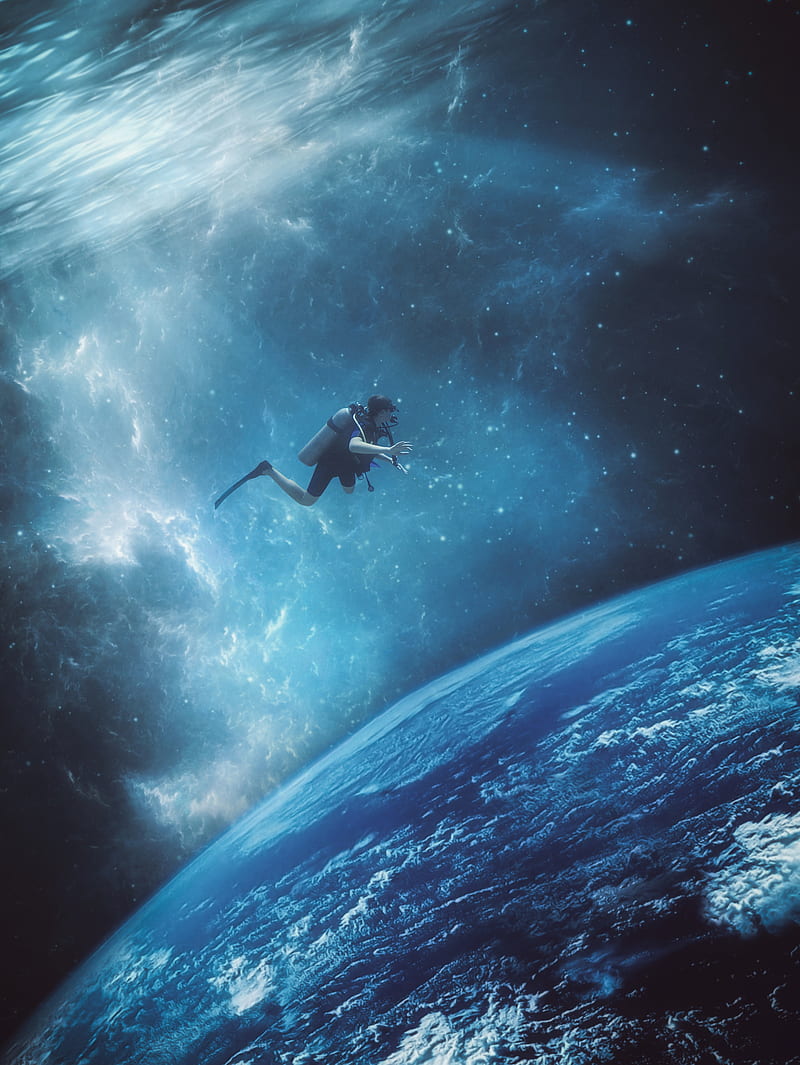In this captivating multi-color digital art piece, we see a vertically rectangular image without a border, blending elements of both deep-sea diving and outer space exploration. The top left corner of the image features the shimmering surface of water, illuminated by radiant, penetrating light rays that suggest an underwater scene. This transitions seamlessly into a cosmic setting with the blackness of space appearing prominently in the lower left and upper right parts of the background, dotted with distant stars and possibly the vibrant gases of a nebula.

Descending from the water surface into the center of the composition is a scuba diver, clad in a black wetsuit with a gray tank and flippers, accompanied by a trail of air bubbles that emphasize his recent departure from the aqueous environment. Despite being poised for a plunge beneath the waves, the diver finds himself suspended in the void of space.

Directly below the diver lies a striking blue planet, shrouded in swirling white clouds. While the planet's identity remains ambiguous, its features bear a resemblance to Earth, with visible continental terrains and oceanic details. The diver, symbolically bridging the realms of sea and space, appears to be gazing contemplatively at this celestial body, blurring the lines between aquatic and astronomical frontiers in a surreal and mesmerizing tableau.